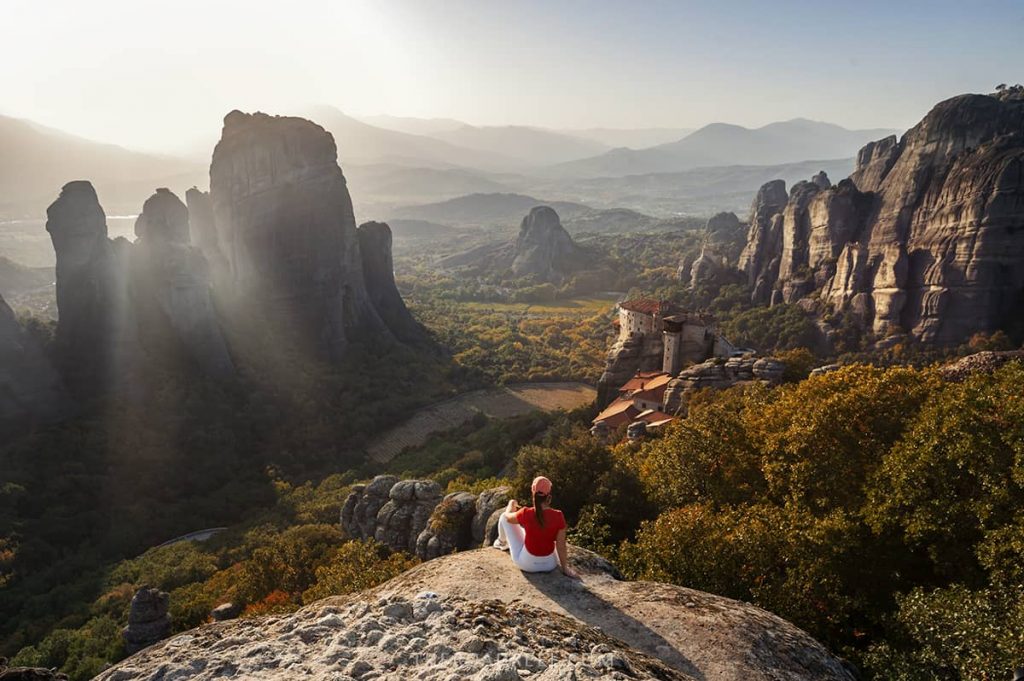In this breathtaking scene of the Midwest, reminiscent of Utah's iconic cliffs and mountains, the centerpiece is a large gray rock. A woman dressed in white pants, an orange shirt, and a pink cap with a ponytail cascading down, sits poised on the rock, gazing ahead meditatively. The camera captures her from behind as she overlooks a valley surrounded by towering rock formations on either side. The sun illuminates the scene from her left, casting an ethereal glow over the beige and tan rocks, and creating muted shades of purple and gray-green in the distance. Sparse greenery and foliage dot the landscape, appearing more yellowy-orange due to the sunlight. Far off in the distance, among the varied heights of the mountains and rock formations, the faint outlines of homes and towns are just visible, blending seamlessly into the natural beauty.